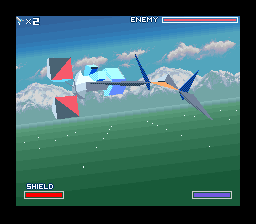This image appears to be a screenshot from an older, low-graphics video game, reminiscent of something from Nintendo or Atari. The scene features two planes in the sky—a detailed plane with grey wings, blue accents, and an orange section, and a larger plane adorned in light and dark blues, whites, greys, and red. Below the planes is a green field that gradually lightens towards the horizon, leading up to snow-capped mountains. The sky above is blue with scattered white clouds. In the top left corner, a label reads "Times 2" next to a ship icon, indicating lives left. The top right corner displays the word "Enemy" with a full red bar showing enemy health status. The bottom left corner features the word "Shield" and a red bar indicating full shield strength. In the bottom right corner, a purple bar shows the player's health. The entire image is enclosed within a black frame.